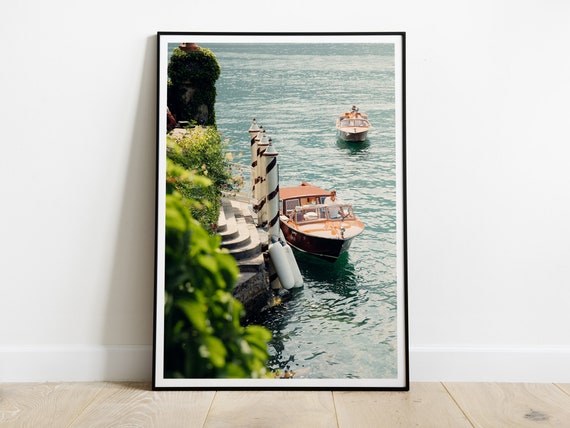This image captures a framed photograph leaning against a very light beige or white wall, which features a slight lip at the bottom. The floor beneath is a light-colored wood, adding to the minimalistic setting with no other visible objects. The thin, black frame of the picture casts a soft gray shadow on the wall, while the picture itself is bordered in white. The photo depicts a serene lakeside scene with two old-fashioned wooden boats, one docked at the forefront and another farther back. The dock features distinctive white pillars adorned with black stripes, resembling barber poles, and leads up to a flight of stairs that disappear into lush greenery on the left side. The water in the image is a tranquil light blue-green, evoking the idyllic charm of a place like Lake Como in Italy. The boat at the forefront is being navigated by a man, adding a touch of life to this picturesque and nostalgic setting.